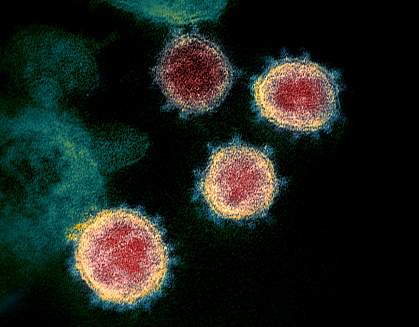The microscopic image showcases a close-up of four circular biological entities, possibly resembling a virus. Each of these entities features a red core, encircled by a yellow band. Extending from these yellow borders are short blue spines. The background is predominantly black, with a blurred, turtle-shaped blue blob on the left side, and some diffused greenish-white elements that add to the grainy texture of the overall image. The image is fairly small and rectangular, lacking any text, numbers, or letters, and despite the graininess, the colors and details are clearly visible. The right side of the background remains completely black, while the left side is more visually complex. One of the entities stands out with a deeper red core but lacks the yellow border prominent in the others.